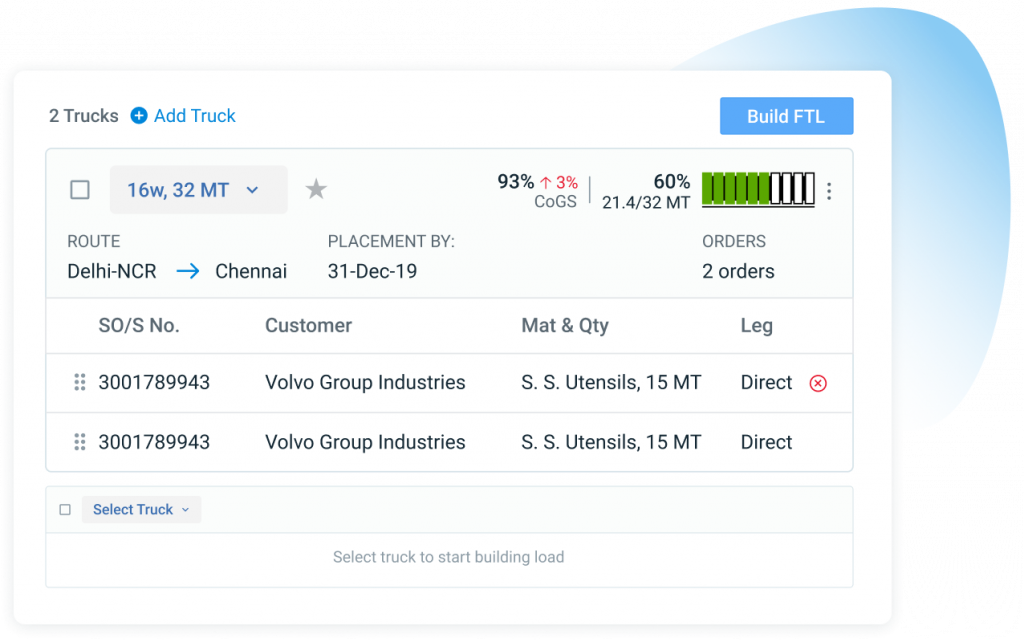In the background, there's a blue hue with two trucks prominently featured. The image includes various geometric shapes such as a circle, square, plus sign, and an unchecked box. A high truck marked with "FTL" is visible. There is a gray square with the text "16MW, 32MT", and a gray star indicating a performance rating of 93%.

The display shows metrics like "21.4 out of 32MT" and "60% battery" or possibly "60% status". The route plotted runs from Delhi-NCR to Chennai, with a deadline for placement by December 31, 2019. An order is directed towards "SLS" and includes the identification number 300178943. This order is associated with Volga Industries, listed as the customer.

Further details mention "man and quantity: SS utensils, 15MT" twice, indicating a shipment of stainless steel utensils weighing 15 metric tons. A directive includes a circle and an "X", with another unchecked box and a prompt to "select truck."

The overall background transitions to white and then gray below with the message “select truck to start building load,” suggesting the commencement of a shipping process. This setup might include dividers, hinting at some organizational structure within the shipping trucks.

This image appears to be a detailed visual representation of a logistics or shipping management system.